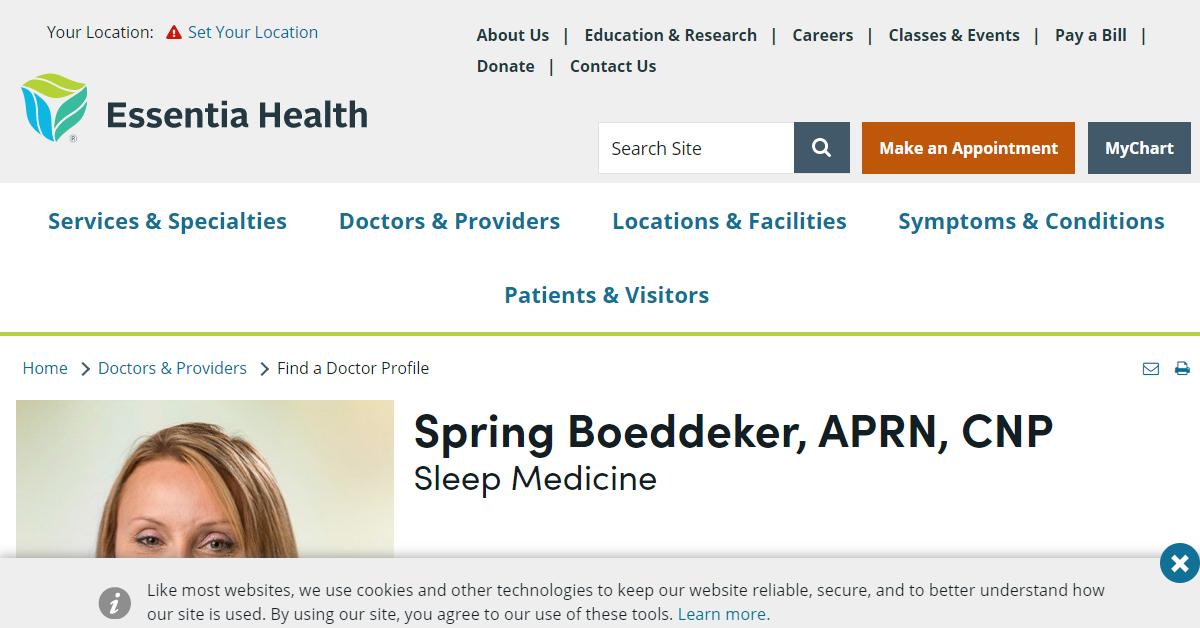The screenshot captures the Essentia Health website interface. At the top of the screen, a gray horizontal bar displays the Essentia Health logo and a series of black text menu items against the gray background. This gray section also includes options such as "Search Site," "Make an Appointment," and "My Site."

Below this, the majority of the screen features a white background. The next prominent horizontal section contains blue text with the following options: "Specialties & Services," "Doctors," "Locations & Facilities," "Symptoms & Conditions," and "Patients & Visitors." A green line separates this section from the rest of the page.

Beneath the green line, a breadcrumb trail indicates the navigation path: "Home," "Doctors & Providers," "Find a Doctor." On the left side, the top part of a profile picture of a Caucasian woman appears. She has dark blonde to light brown hair and is looking directly at the camera; the visible section of the image only reveals up to just below her eyes.

To the right of the image, large black text reads "Spring Boudicca, APRN, CNP." Below her name, in smaller text, it states her specialty: "Sleep Medicine." 

At the very bottom of the screen, a gray cookie disclaimer bar is visible, featuring a blue 'X' button for closing the notice.